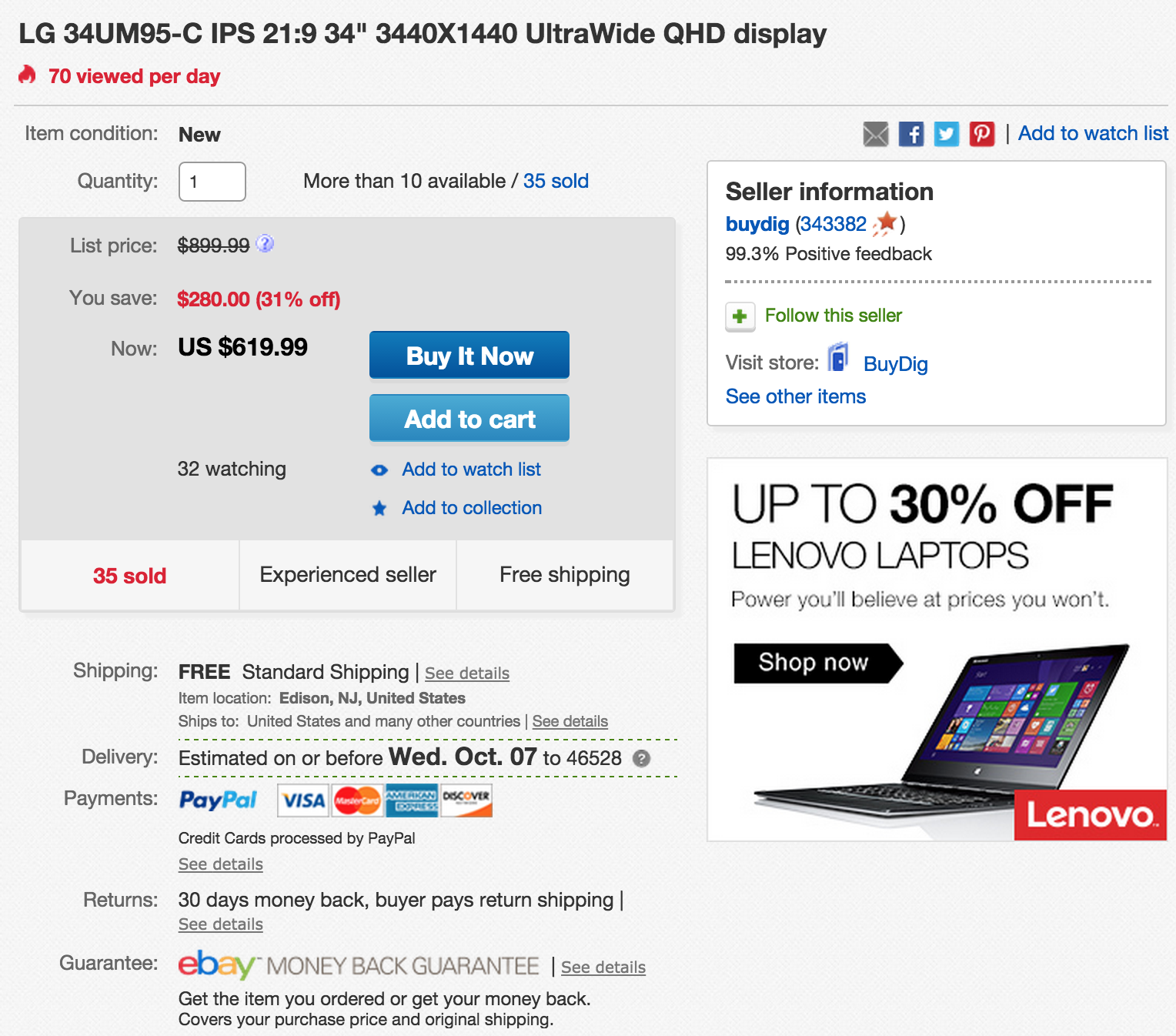Capturing the essence of a bustling online store, the image showcases a prominently featured product at the top left: the LG DDR4-UM95C IPS2129, a 34-inch ultrawide QHD display with a resolution of 3440x1440. The product experiences high visibility, garnering an impressive 70 views per day. Detailed information about the item is included, such as its Condition (New), Availability (More than 10 available), and Sales Record (35 sold, depicted in vibrant blue text). The list price of this premium display is $899.99, but it's generously discounted by 31%, bringing the price down to $619.99, highlighted in bold red.

The interface provides user-friendly options with two buttons on the right side: a blue "Buy It Now" button, and a slightly lighter blue "Add to Cart" button. Additional features include a blue tag offering options to "Add to Watch List" and "Add to Collection." Notably, "35 sold" is reiterated in red on the bottom left. The benefits of purchasing this item are highlighted with mentions of an "Experienced seller" and "Free shipping."

Further down, the shipping details specify "Free standard shipping," with the item located in the United States and shipping available to many countries. Delivery is estimated between Wednesday, October 7th and Friday, October 9th. Payment options are diverse, including PayPal, Visa, Mastercard, American Express, and Discover, all processed by PayPal. The store offers a 30-day money-back return policy where buyers pay for return shipping and backs their sales with the eBay Money Back Guarantee.

On the right, the seller information stands out, with the seller "buydig" boasting a positive feedback score of 99.3%. Options to follow the seller or visit their store are conveniently provided. Below the main product listing, there's an advertisement for Lenovo laptops, promising up to 30% off, with a call to action to "Shop Now." The Lenovo logo, displayed in white against a red background, is positioned at the bottom right to seize attention.

This image embodies a seamless online shopping experience with clear visuals and comprehensive information, designed to engage and inform potential buyers effectively.